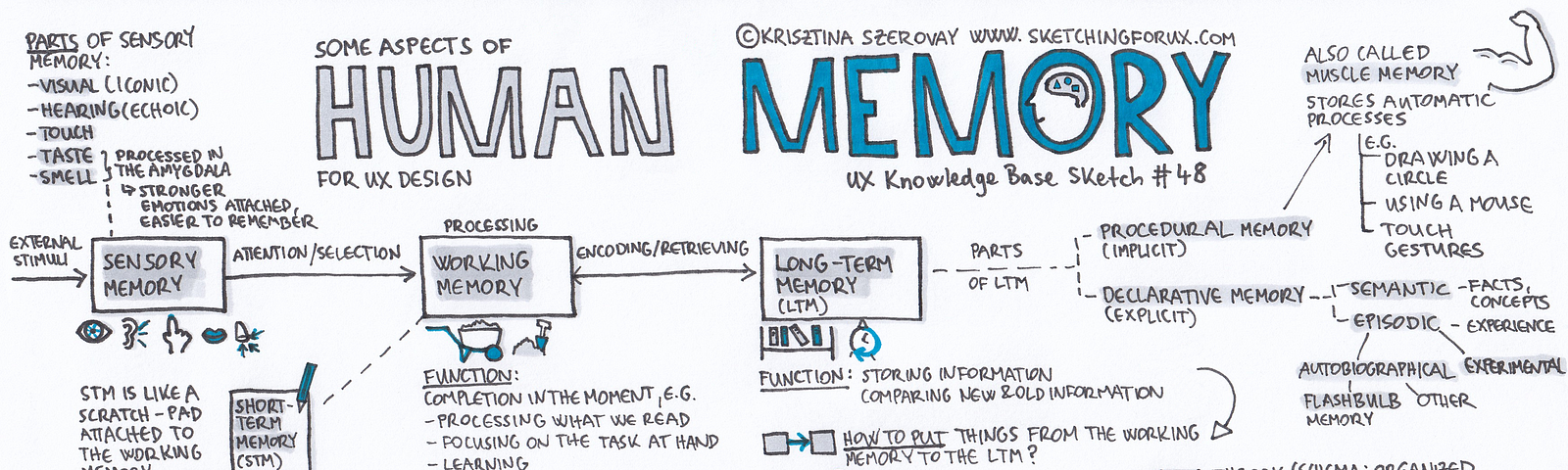The image is a detailed educational chart titled "Some Aspects of Human Memory for UX Design" and labeled as "UX Knowledge Base Sketch Number 48" by Christina Severo, with a web address for more information listed as www.sketchingforux.com. The chart meticulously outlines the flow of human memory, starting with sensory memory, which processes inputs like visuals (iconic), sounds (echoic), touch, taste, and smell. It progresses to working memory and then diverges into long-term memory, which is categorized into procedural (muscle memory), declarative memories, and other subdivisions. Each section of the diagram includes descriptive text boxes and relevant imagery, offering detailed explanations of the functions and processes associated with different types of memory.